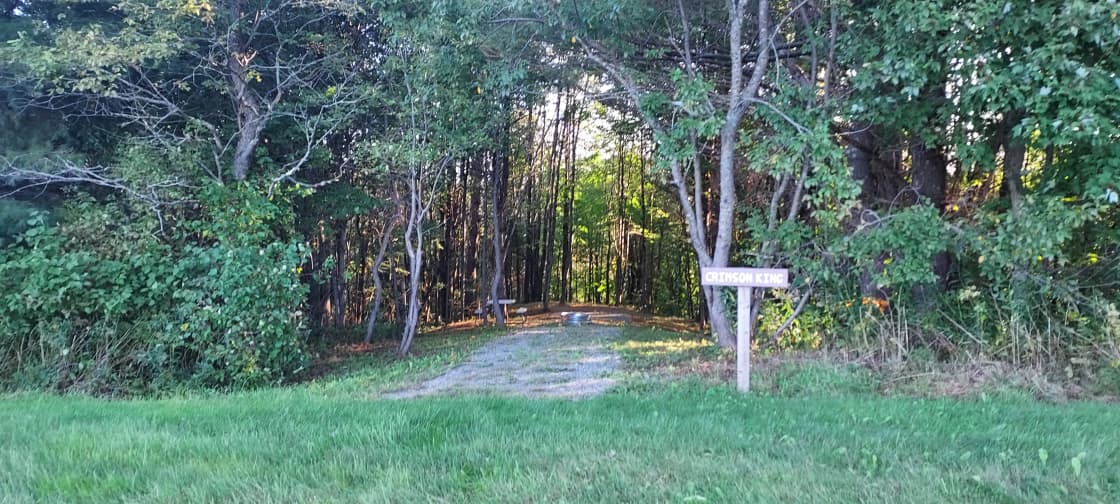The image features a serene woodland scene with towering trees flanking a central dirt path. The path, primarily composed of grayish-brown soil with sparse grass patches, stretches ahead through the dense forest. In the foreground, the path opens up into a verdant area covered in lush green grass. 

Prominently, a wooden signpost stands at the entrance to the path. The post is designed with a vertical beam supporting a horizontal bar, which bears the inscription "Crimson King" in bright yellow letters. Just at the mouth of the path, a puzzling silver object rests on the ground, its exact purpose or identity remaining ambiguous. 

Further into the forest, another sign can be faintly discerned on the left side, adding an element of mystery and inviting curiosity about the hidden narratives within the woods. The tall trees lining the path create a natural archway, guiding the viewer's eye deeper into the tranquil, inviting forest scene.